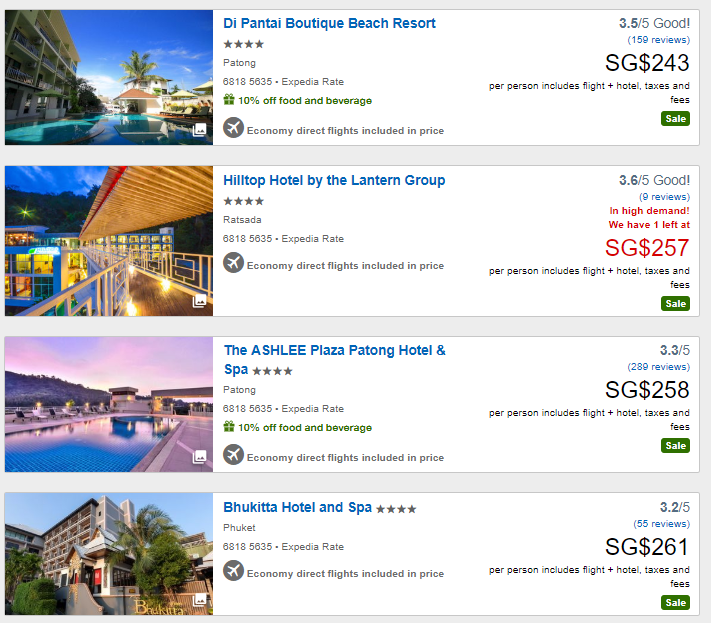Here is a detailed and polished caption for the image:

---

Explore Exquisite Hotel Destinations:

1. **Duponte Boutique Beach Resort**: Featured at the top, this luxurious hotel, showcased with a stunning image of its inviting swimming pool, boasts a 3.5-star rating from 159 reviews. Priced at SG$243, it includes economy direct flights, making it a great value destination.

2. **Hilltop Hotel by the Lantern Group**: This destination is highlighted with a captivating photo of a clear blue sky and an outdoor hallway. Priced at SG$257, it offers a serene and picturesque stay.

3. **A. Schley Plaza Patong Hotel and Spa**: Illustrated with an impressive image of a large swimming pool, this hotel is priced at SG$258 per person. The offer includes both flights and hotel taxes and fees, ensuring a hassle-free experience.

4. **BHUKI TTA Hotel and Spa**: The fourth entry in the list, this hotel offers an exceptional experience with a four-star rating. Priced at SG$261, it promises comfort and luxury for discerning travelers.

---